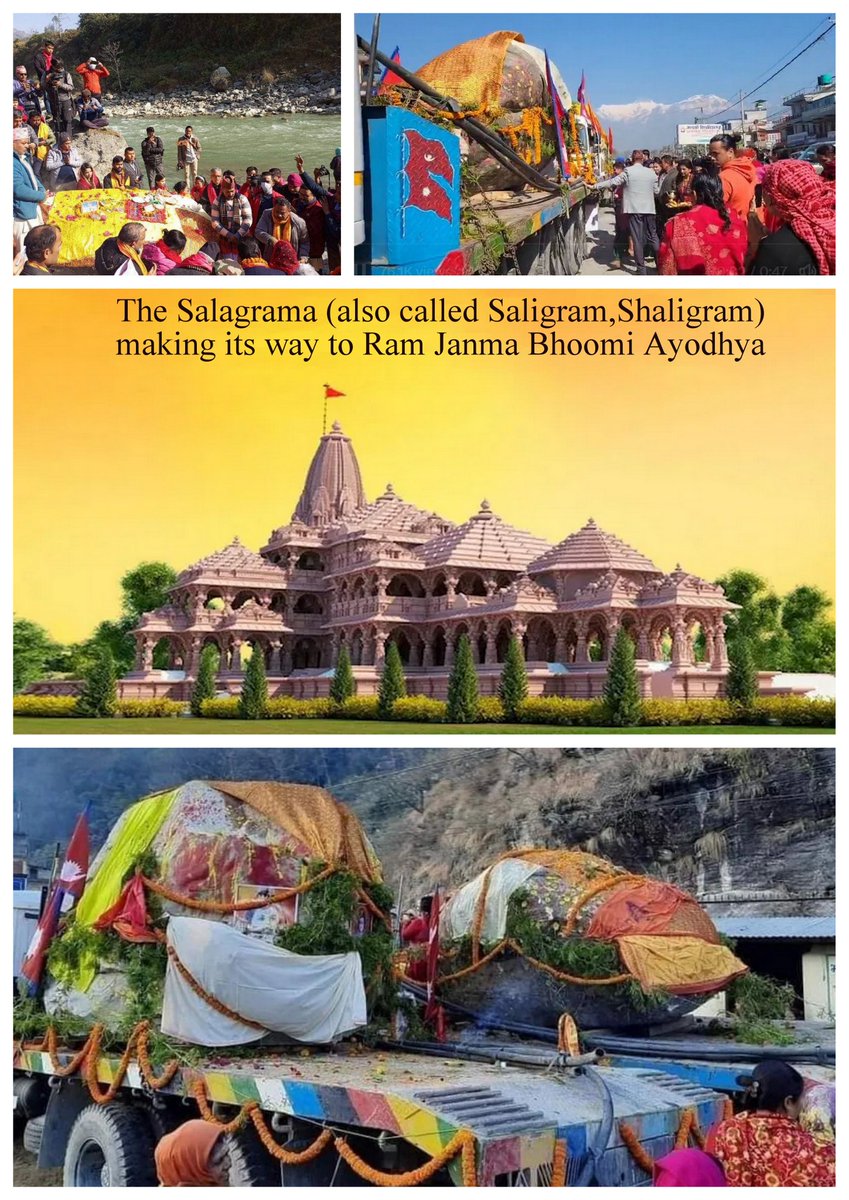The vertical rectangular image is a composite of several photographs, focusing on a culturally significant event. At the top, two photographs show groups of people gathered around a platform, suggesting a communal activity, likely in Southeast Asia. The middle section features the main text, on a gold background, which reads, "The Saligrama, also called Salagram or Shaligram, making its way to Ramjanmabhumi Ayodhya." Below the text is an image of an impressive ancient structure, resembling a palace with pagoda-shaped tops and an open bottom floor, indicative of Indian architectural style. The bottom photograph shows an item, covered in tarps, being transported on the back of a flatbed truck, likely part of a float in a parade.